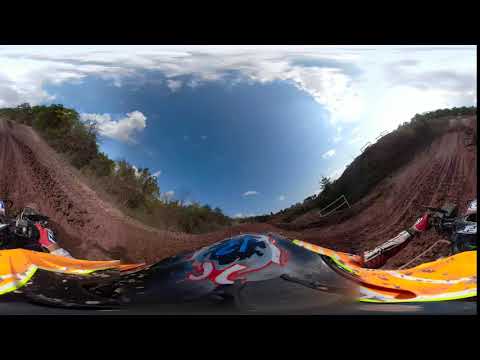The image captures an outdoor dirt track framed by the handles of a four-wheeler, suggesting it was taken from the rider's perspective. The scene showcases a hilled track that dips into a valley and rises again, bordered by grass and brush. The foreground reveals distorted orange elements, possibly the vehicle's hood or a jacket. The dirt pathway features a mix of brown shades and seems to have a unique design on a central hump, including a blue circle with a black image inside and a red swoop reminiscent of a mustache. On either side of the track, the orange coloring contrasts vividly. Above, a striking blue sky is dotted with clouds, particularly dense towards the top, adding a sense of depth to the panoramic view. The colorful details of the four-wheeler—yellow, blue, red, and black—add to the dynamic composition of the image.